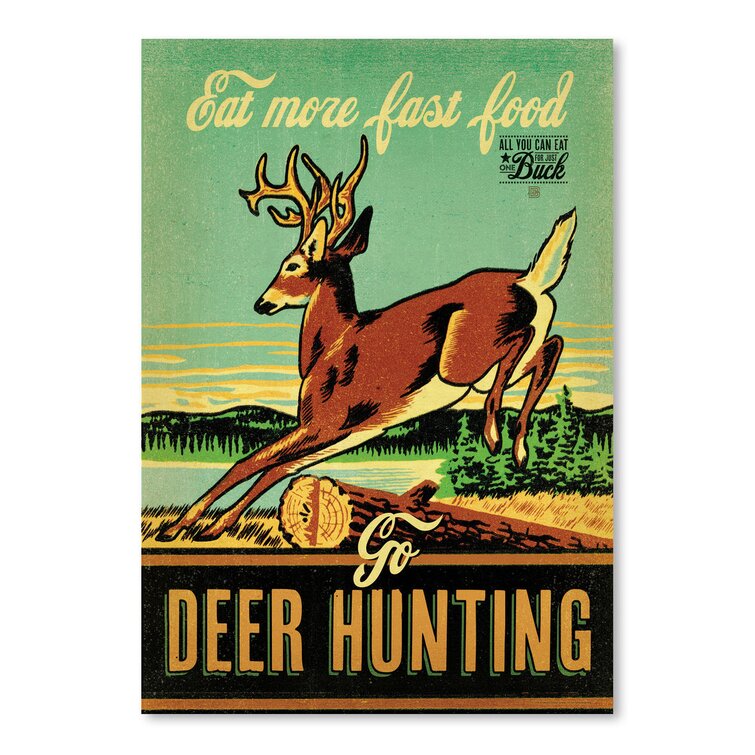The poster features a cartoonish drawing set against a scenic nature backdrop, with a blue sky streaked with yellow, a serene lake, evergreen trees, and distant mountains. A prominent white-tailed deer with impressive antlers is captured mid-leap over a fallen log. The foreground includes patches of brown grass, further enhancing the wilderness theme. At the top, in elegant cursive white font, the slogan "Eat more fast food" stands out. Below this, a distinct black stamp-like section declares, "All you can eat for just one buck." Centered beneath the image, the word "Go" appears in white cursive, set against a brown strip that transitions into a black background. Bold, beige-colored, printed letters spell out "Deer Hunting," completing the poster's rustic, adventurous vibe.